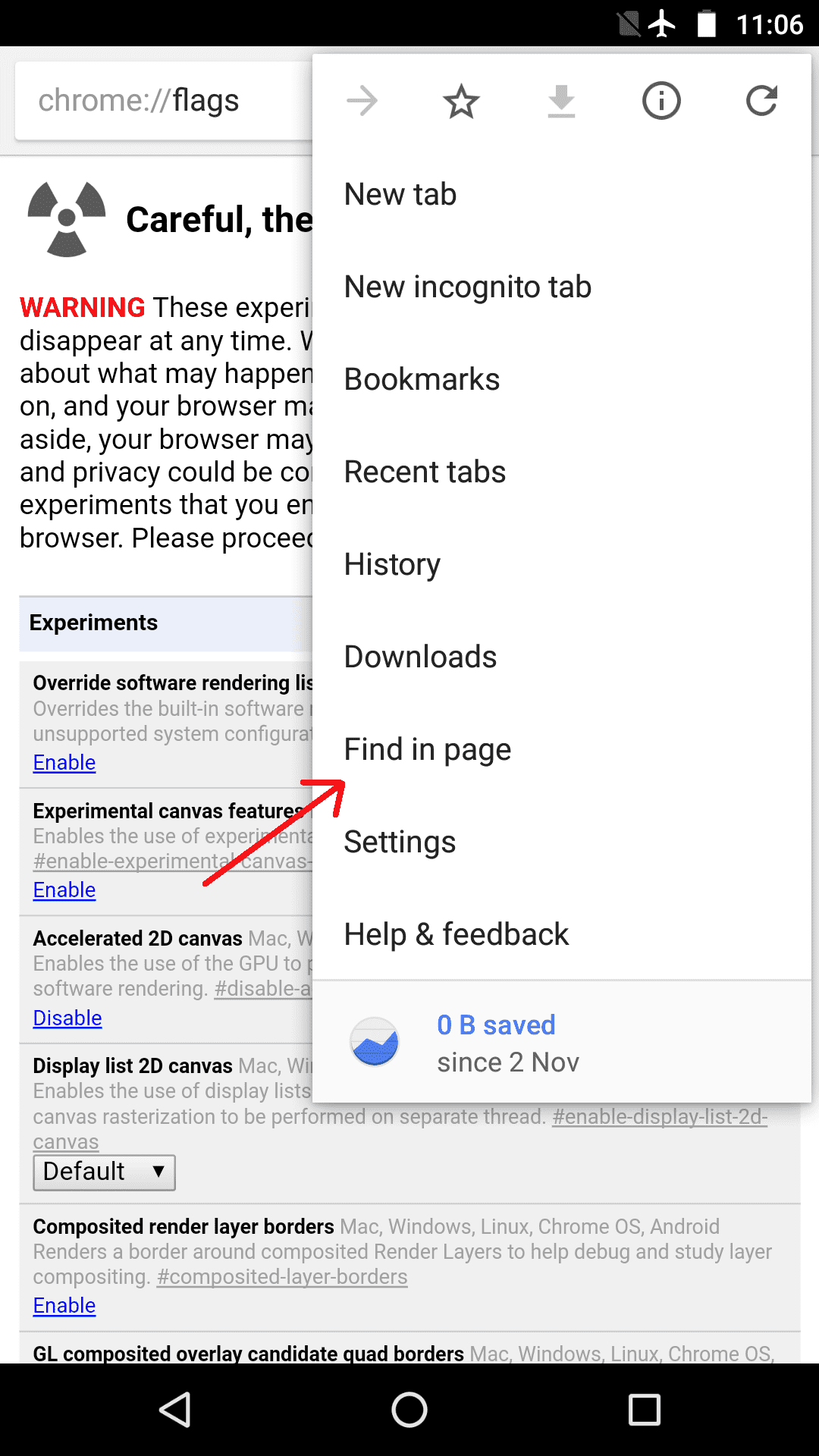The image displays a complex GUI layout, primarily featuring different user interface elements of what appears to be a browser settings or experimental features panel. 

At the top, there's a solid black rectangle serving as a header. On the right-hand side, a gray document icon with a diagonal line through it is visible. Directly underneath this is a white rectangle symbolizing an airplane, labeled with the number "1106."

Below this section, a gray-outlined rectangle is present, containing several icons and labels. On the left side, an arrow pointing right is adjacent to a star icon, followed by an arrow pointing downwards and a line beneath it. Additionally, there is a circle with an "i" in its center and another circle featuring an arrow.

Within this gray-outlined rectangle, various menu options are listed: "New Tab," "New Incognito Tab," "Bookmarks," "Recent Tab," "History," "Download," and "Find In Page," the last of which is highlighted by a red upward-pointing arrow. Additional menu options include "Settings" and "Help and Feedback."

Further down, there's a small gray rectangle housing a slightly darker gray circle with blue hills inside, showing "0B Saved" in blue, and a timestamp "Since 2 NOV". 

Adjacent to this is another gray rectangle partially obscured by the white rectangle above. It contains a URL prefix "chrome://," an item labeled "flags" in black, and a warning symbol followed by the text "Careful, the" partially hidden behind the white rectangle. Beside this, there is a warning message in red, "Warning," followed by a block of black text, also partially obscured.

Towards the middle of the image, a blue rectangle with the text "Experiments" and several gray-outlined rectangles convey different experimental features, including "Override Software Rendering," "Experimental Canvas Features," each accompanied by blue, underlined "Enable" links, and gray descriptive text. One notable feature, "Accelerated 2D Canvas," has a red arrow pointing to it and the "Find In Page" menu option.

Continuing further down, another segment includes terms like "Display List 2D Canvas" with a blue underlined "Disable" option, and additional descriptive text mostly hidden by the white rectangle. There's also a gray-outlined rectangle labeled "Default" with a downward-pointing arrow, "Component Render Layer Borders" followed by more descriptions in gray, and another blue underlined "Enable" link.

At the very bottom, another black rectangle includes a trio of symbols: a left-pointing triangle, a circle, and a square, possibly controlling playback or navigation functions.